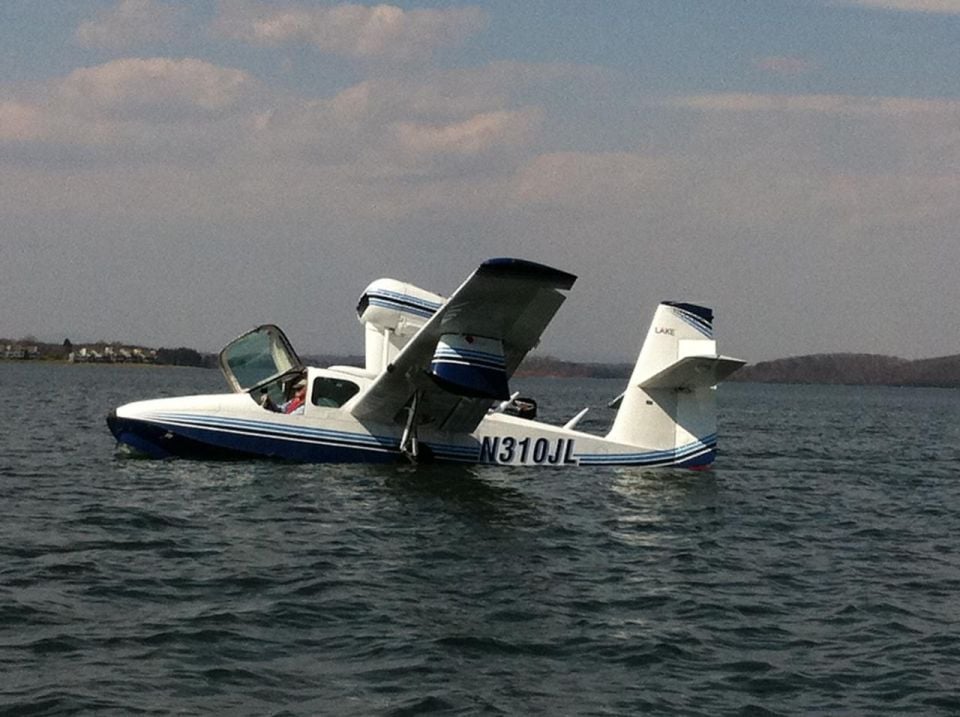The photograph captures a striking scene of a white aircraft with a dark navy blue underbelly, adorned with light and dark blue stripes on its sides and wings, floating on a body of water. The plane, which has the registration N310JL prominently displayed, also bears the word "Lake" on its tail fin, indicating it's designed for water landings. The aircraft's door is popped open, revealing a gentleman in a red coat and hat, seated in the cockpit. The choppy, dark water adds drama to the scene, contrasting with the clear blue sky, dotted with fluffy white clouds. In the distant background, rugged brown mountains and what appears to be a small settlement on the far shore complete the picturesque landscape. The plane, central to the photo, appears to have just landed smoothly on the water, rather than crash-landed, as evidenced by its intact state and the pilot's calm posture.